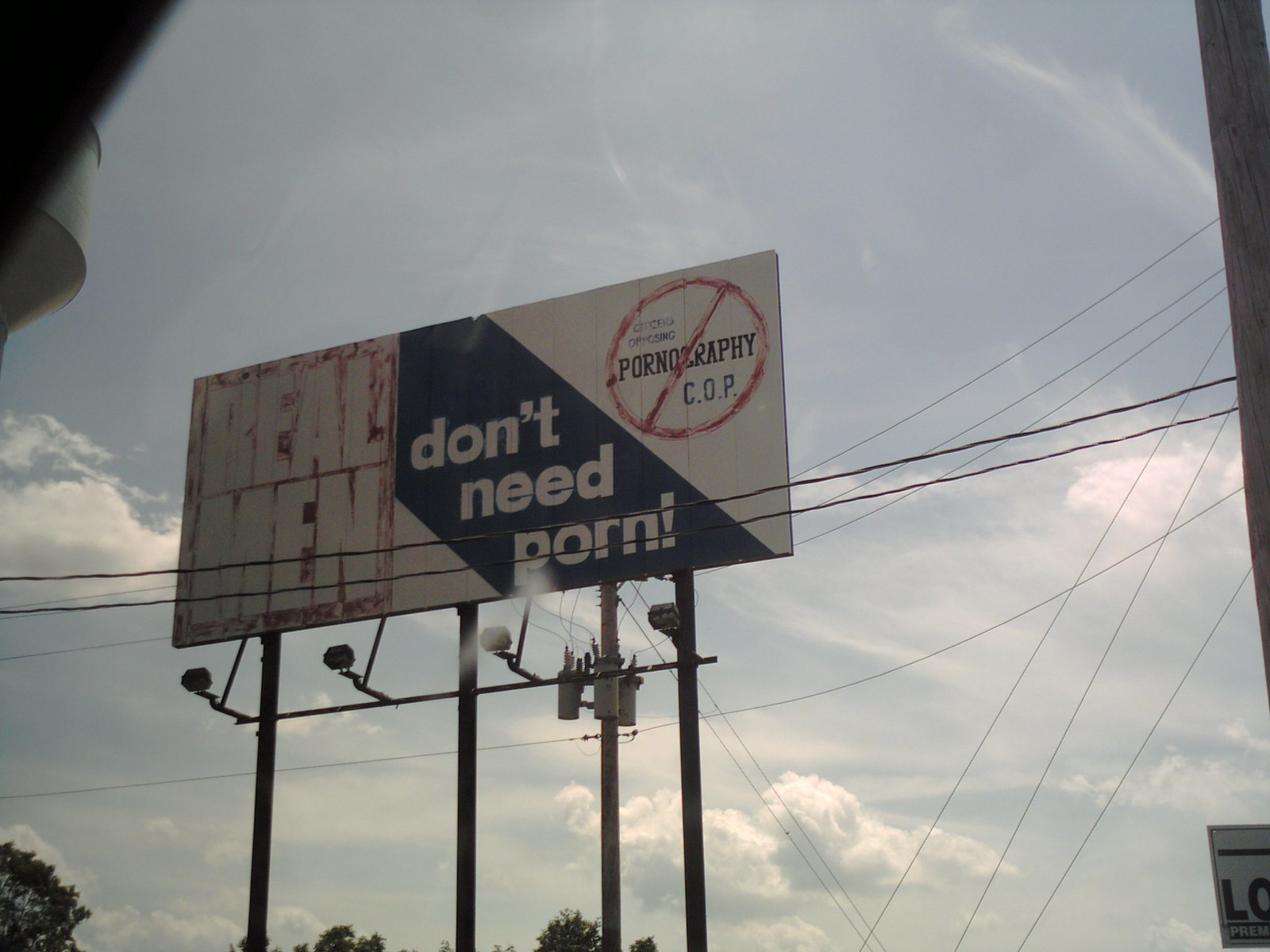This photograph captures an outdoor billboard against a bright blue sky, taken from a low angle looking upward. Dominating the center of the image, two power lines traverse downward, partially obscuring a white billboard situated atop four metal poles that emerge from the middle left of the frame. The billboard, positioned prominently in the middle part of the image, features a slanted blue stripe with white text that reads "Don't Need Horn." In the top right corner of the billboard, a red circle with a slash through it encloses the word "Pornography," accompanied by the letters "C.O.P." in black. At the base of the billboard are four upward-pointing lights, presumably for nighttime illumination. The overall scene is bright, suggesting the photograph was taken during daylight hours, and the top edges of some trees can be seen at the bottom of the image.